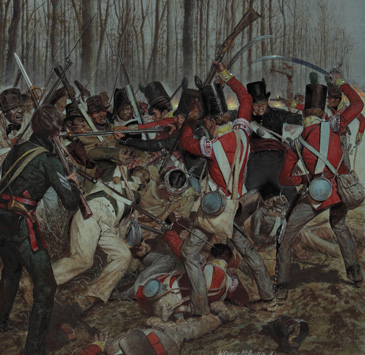The image depicts an intense battle scene, possibly a painting, rendered with meticulous detail. On the right side are soldiers clad in red uniforms, reminiscent of the Revolutionary War-era Redcoats, while their adversaries on the left don blue and brown uniforms, with some in tall top hats of varying heights. They're engaged in fierce melee combat, brandishing swords, sabers, cutlasses, and bayonets, with soldiers being stabbed, thrown down, and struck over the heads with muskets. The foreground highlights the chaos, showing a man on the ground amidst the fray, and another close by, while a soldier in a bluish-green uniform looks on, gun in hand. The background features a stand of thin, leafless trees, creating a stark, late fall or winter atmosphere, under a dark, hazy blue to gray evening sky.